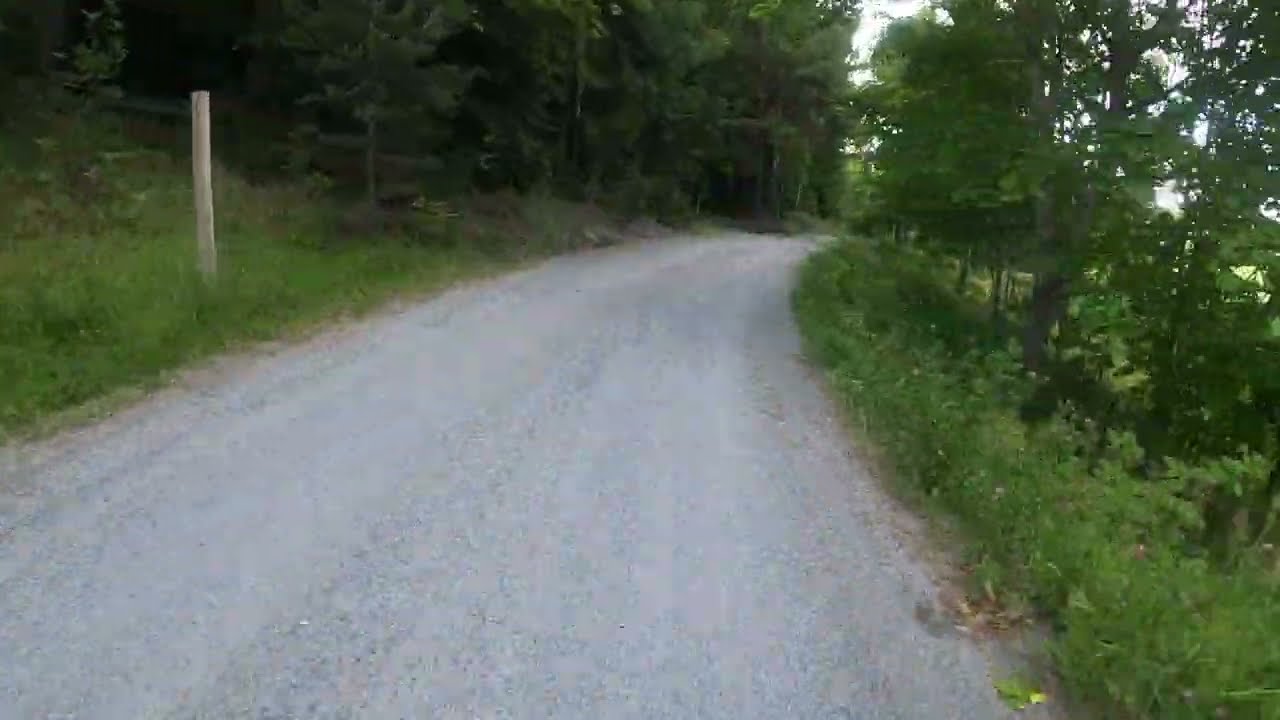The image showcases a serene countryside scene featuring a light gray gravel road that curves and disappears into a lush, wooded area. Tall, unkempt grass flanks both sides of the road, which is wide enough for a car and lined with patches of dirt and scattered leaves. Various thin trees with green leaves and a mix of evergreen and deciduous trees frame the road, enhancing the natural feel. On the left side of the image, a solitary truncated wooden pole stands out against the verdant backdrop. The sky overhead is a light gray, clouded and sunless, suggesting an overcast day. The road curves into the distance, obscured by the dense foliage, imparting a sense of mystery and tranquility to the scene.